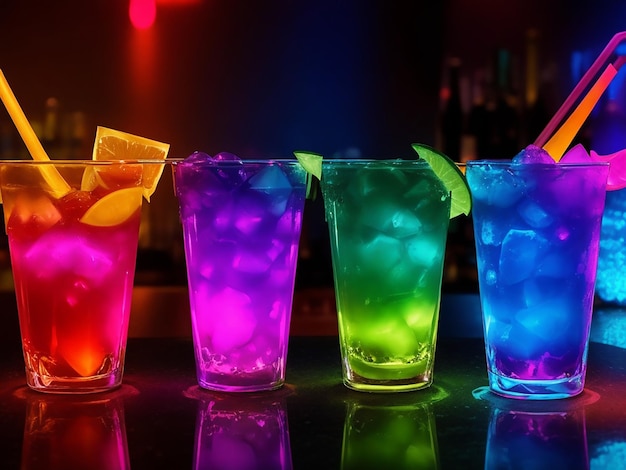This professionally taken photograph showcases a sleek, dark gray bar setting with a blurred background hinting at vaguely discernible shelves and bottles. Lined up on a reflective table are four identically shaped glasses, each containing a vividly colored drink. Starting from the left, the first drink is a vibrant pink, adorned with an orange wedge and an orange straw, featuring some ice cubes within. The second drink presents an ombre effect, transitioning from blue at the bottom to a light purple at the top, and it is garnished with a lime wedge. The third glass holds a drink that transitions from blue to yellow, also topped with a lime wedge and ice. The final glass on the right contains a deep purplish-blue liquid with an orange straw and ice. The drinks are brightly lit, showcasing their rainbow neon hues, giving off a festive and inviting vibe, suggestive of a promotional image for a bar or restaurant.